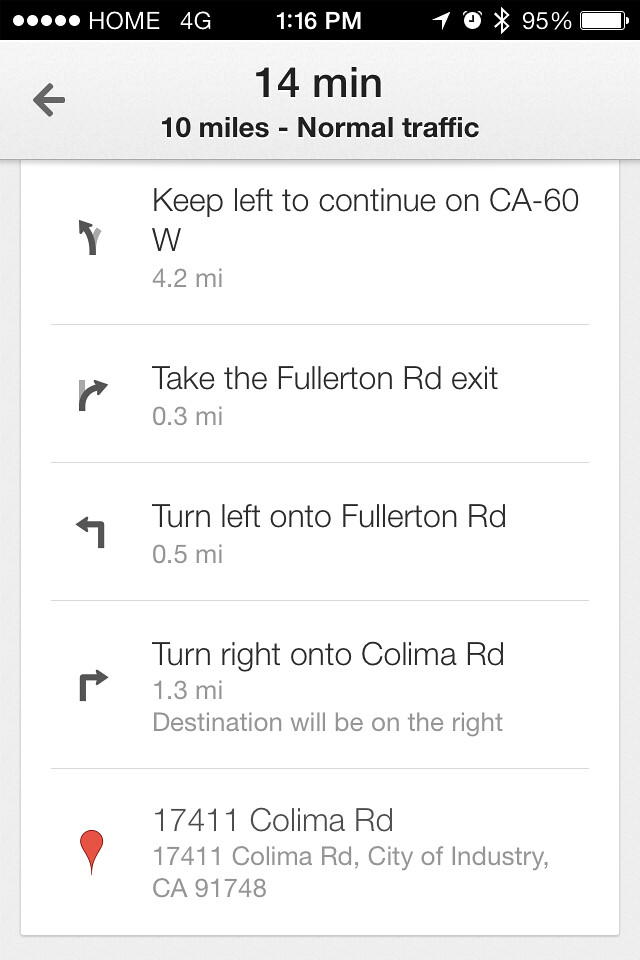The screen displays GPS navigation information on a mobile phone. The map outlines a route that will take approximately 14 minutes to cover a distance of 10 miles, under normal traffic conditions. The journey proceeds on California Highway 60 West, then exits onto Fullerton Road, and continues with a right turn onto Colima Road, leading to the final destination in the City of Industry, California. This city is colloquially known as "Colima." The current time is 1:16 PM, the phone battery is at 95%, and it is utilizing a 4G network. The interface presents this information on a clean white background with thin black font.